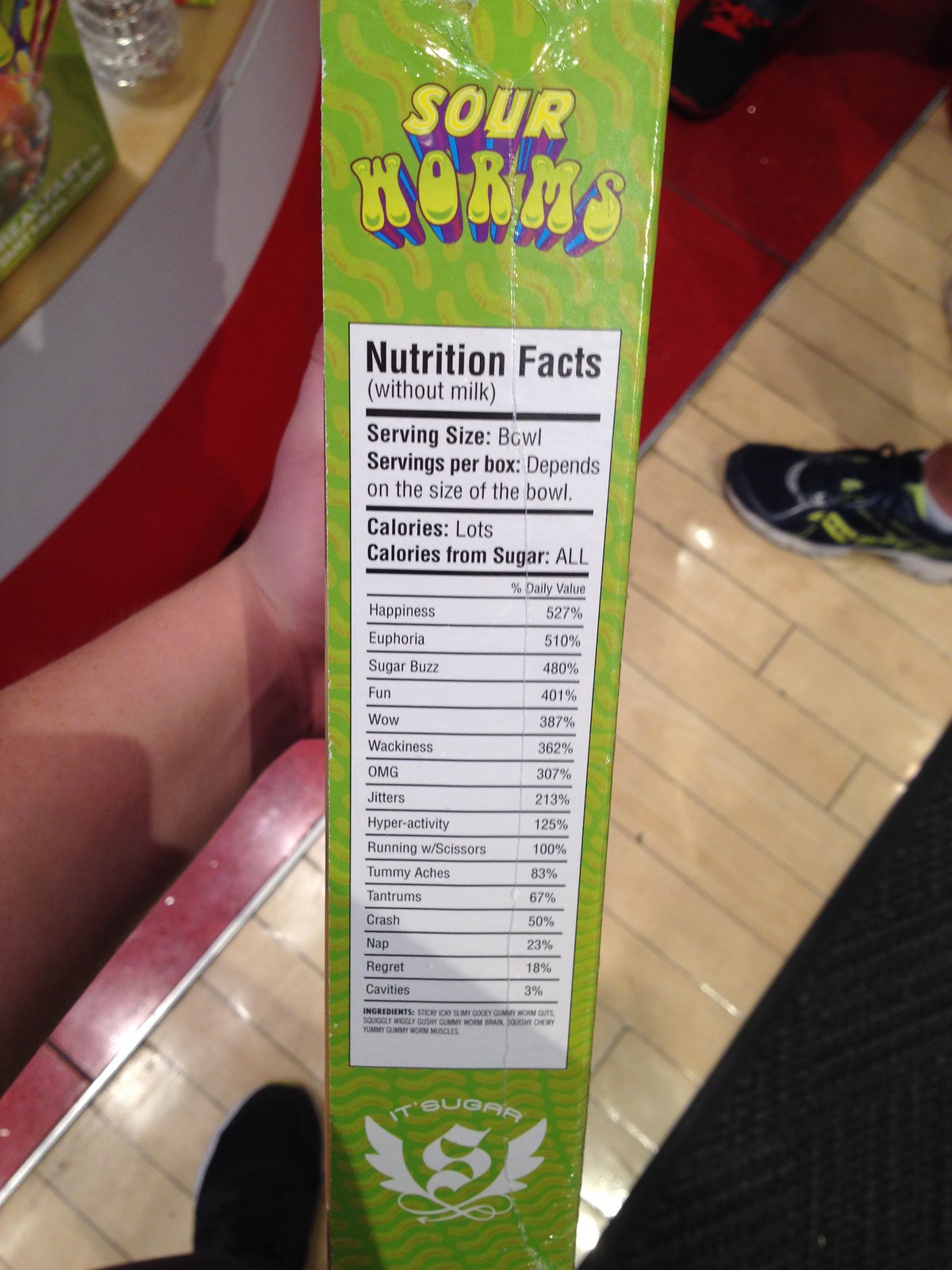This photograph appears to be taken inside a store and features a close-up of a bright green cereal box prominently displaying its nutritional facts. The box is held by a young boy whose left hand is visible in the frame. The box has neon green detailing shaped like worms, and the top portion has "Sour Worms" written in bubble font. Beneath the nutritional facts, there is a stylized logo with an "S" flanked by two feathers or wings and some scrollwork underneath.

The background of the image is divided into three distinct diagonal sections. The bottom left corner has a triangle of black carpeting, typical of commercial spaces. Adjacent to it is a strip of pale pine-colored plank flooring. The top left corner features a bright red vinyl or tile floor. A white display unit with a wood-effect top is visible in the upper left corner, with another green box, potentially the same product, standing on it.

Additionally, a black shoe is noticeable in the bottom left corner, likely belonging to the boy holding the box. Another person’s shoe is partially visible on the right side of the image.